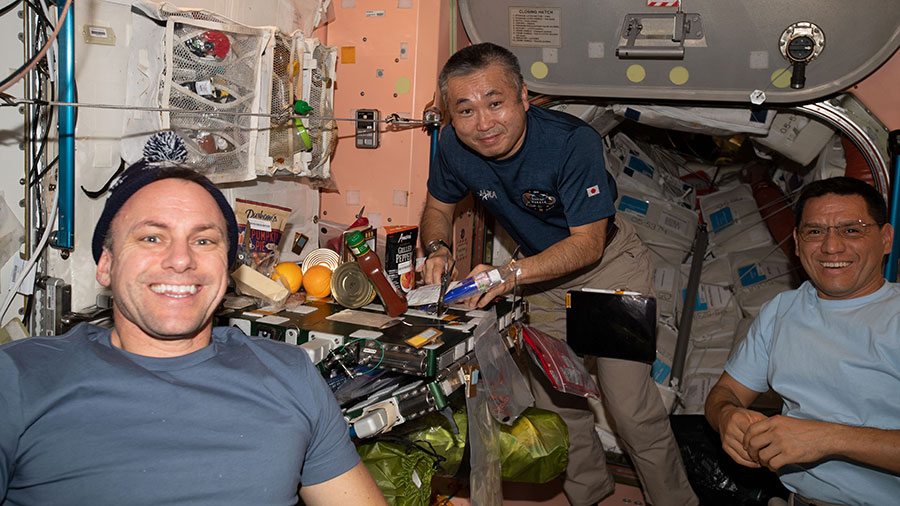The image depicts three men who appear to be in an environment consistent with an International Space Station or another similar space habitat. All three men are smiling and seem to be in good spirits. The man on the left is visible from his chest up, wearing a gray short-sleeved shirt and a knit cap, estimated to be in his 40s, with an outstretched arm that’s partly out of the photo. The middle man, who is hunched over a table or workbench, wears a darker blue shirt, khaki shorts, and emblems on his bicep and chest. He is surrounded by some food items, including a bottle of ketchup and oranges, which appear to be resting on hardware components, adding to the disarray. The man on the right, wearing a light gray short-sleeved shirt and glasses, completes the trio. The background includes various storage compartments, netted areas filled with bags and other materials secured by ropes, consistent with zero-gravity conditions where loose items float. Several pieces of computer equipment, including motherboards and processors without attached monitors, are visible near the men, reinforcing the impression of a technical or laboratory-like setting. Despite the apparent clutter and floating objects, the scene radiates a sense of camaraderie and joy among the three men.